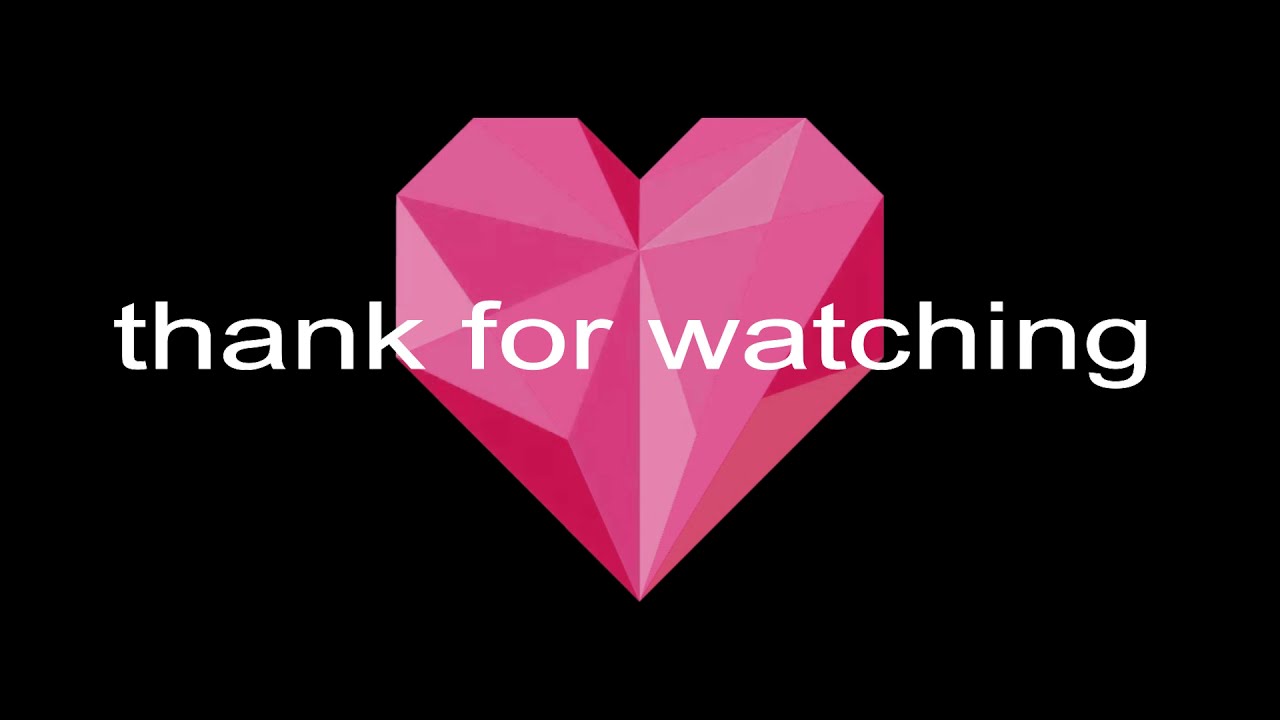The image features a striking, computer-generated, crystallized pink heart at its center, set against a stark black background. The heart is composed of geometric shapes, including squares and triangles, giving it a rigid, angular appearance rather than smooth curves. The heart showcases a spectrum of pink tones, ranging from light pink to almost white, alongside touches of red. Centered across the heart in thin, lowercase white letters is the phrase "thank for watching." The simplicity of the design, with its black background and vivid heart, makes the colors pop, creating a visually appealing contrast. This image appears to serve as a closing slide for a video, such as a YouTube clip, podcast, children's cartoon, or even a movie, intended to thank viewers for their attention despite the grammatical error in the text.